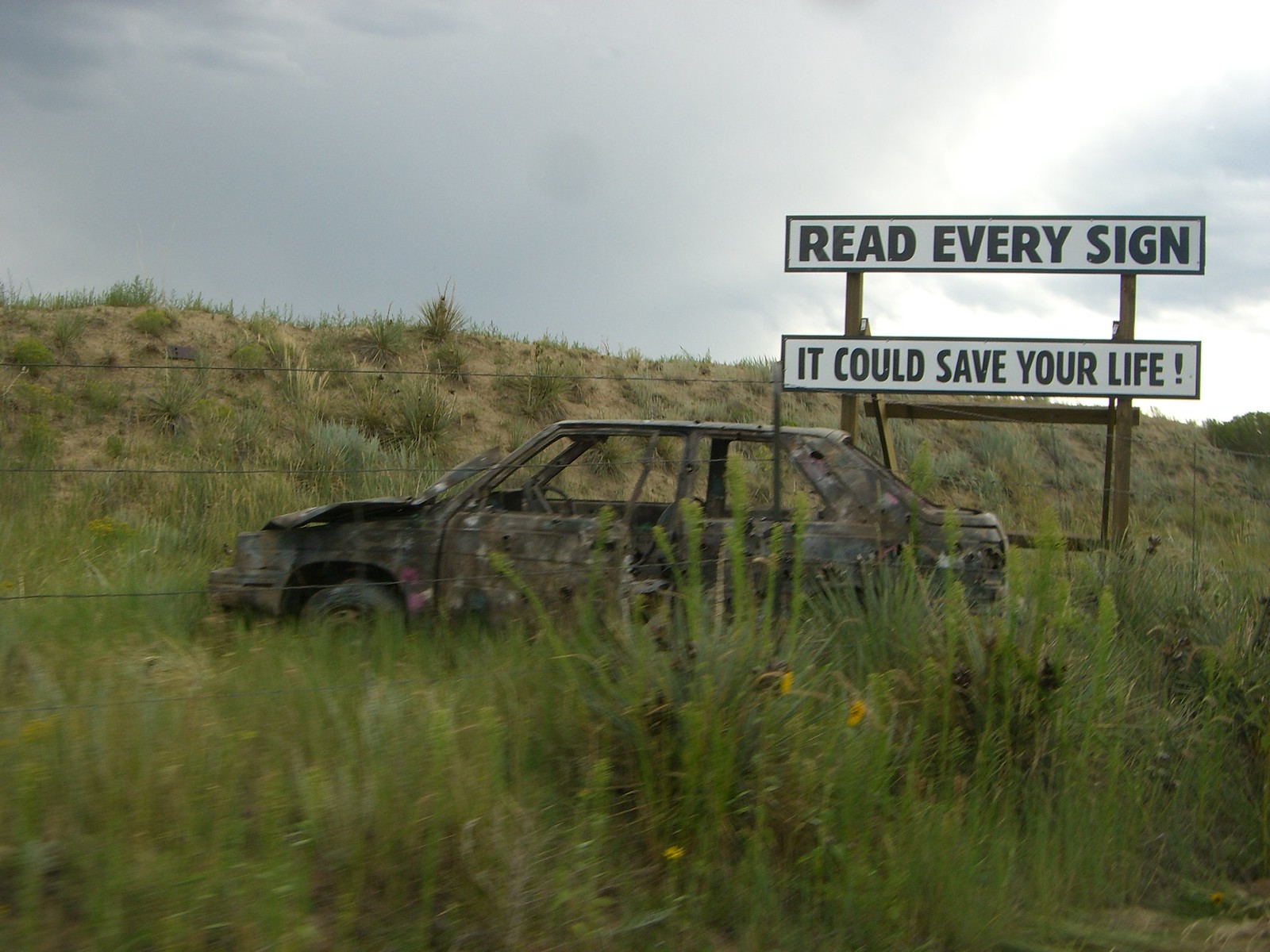The photograph captures a desolate outdoor scene under a gloomy, overcast sky filled with gray clouds, with a faint glimmer of light peeking through on the right side. In the foreground stands a stark, white sign with bold, black lettering that reads, "Read Every Sign. It Could Save Your Life!" This sign is positioned in front of a severely rusted and burnt-out car, devoid of windows and with its doors open. The car bears significant damage, notably a crumpled hood, indicating it has been abandoned for a long time. This scene is set against a backdrop of a small, brown hill adorned with sparse green plants, patches of long wild grass, and yellow wildflowers in a seemingly neglected field. The entire composition suggests a cautionary tale, implied by the juxtaposition of the distressed vehicle and the ominous warning on the sign.